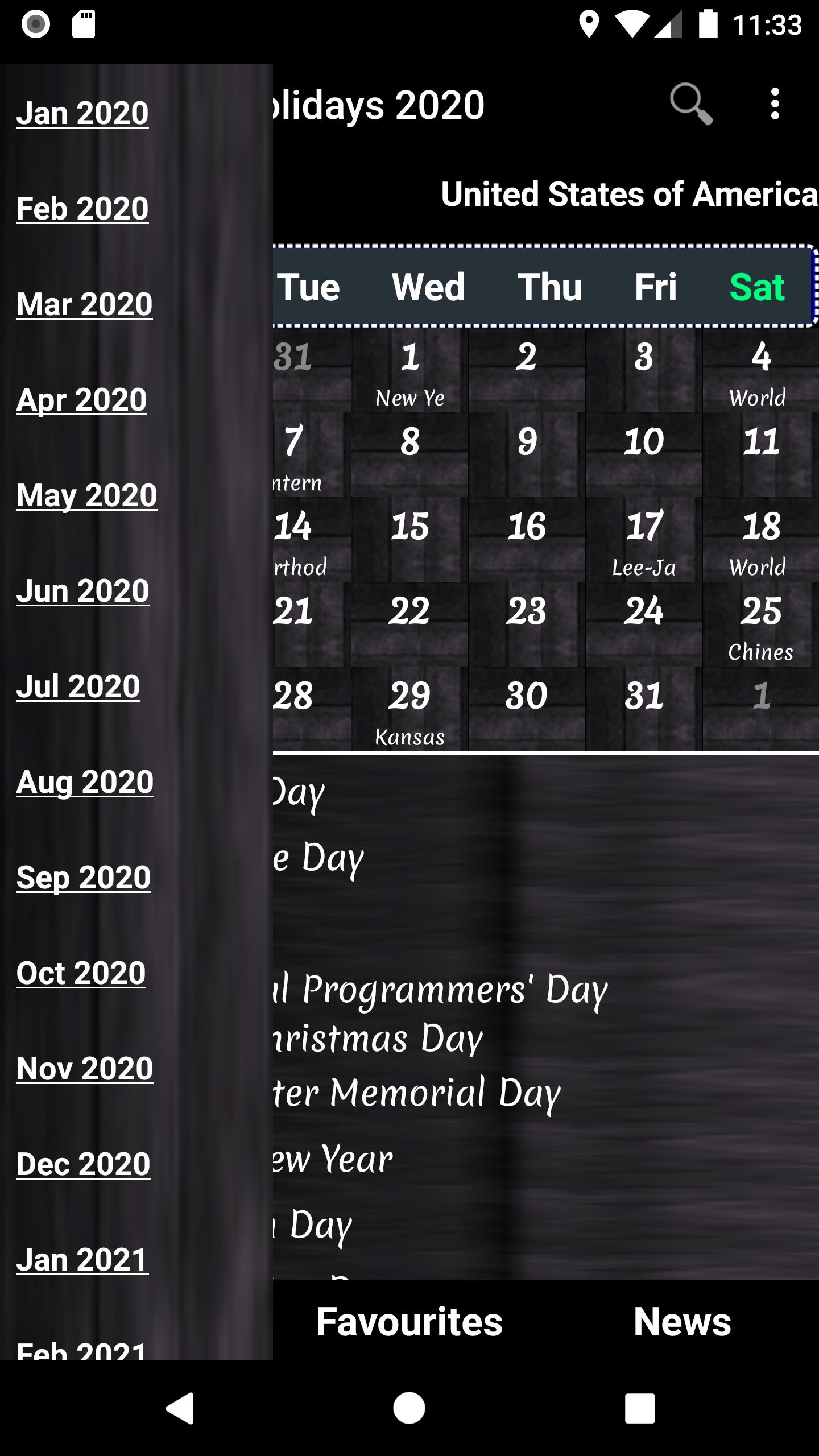The image depicts a smartphone screen displaying a calendar application. In the top-right corner, various status icons are visible, including the Wi-Fi signal indicator, battery percentage, and the current time, which reads 11:33. Just below these icons, a search bar is present. The main content area of the screen shows a calendar for a particular month in the year 2020.

On the left-hand side of the screen, a grey vertical banner lists each month from January 2020 through February 2021, indicating that they are selectable options. The current month displayed on the calendar appears to have 31 days, suggesting it might be January. The days of the week are labeled, with Saturday standing out in green text, whereas Tuesday, Wednesday, Thursday, and Friday are shown in white. Due to the vertical banner obscuring part of the calendar, Sunday and Monday are not visible.

Several days on the calendar have notations beneath them, indicating significant holidays or events such as "World," "China's New Year," and "Kansas," which are specific to various regions worldwide. The calendar also highlights typical American holidays throughout the year.